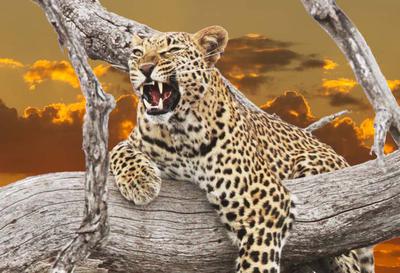The image captures a close-up of a wild cat, either a leopard or jaguar, lounging on a weathered, gray tree trunk with branches extending behind it. The cat, with its distinctive yellowish-white fur adorned with black splotches, is in a semi-reclining position, draped over the log. Its left paw hangs over the front, while the right paw rests on top, supporting its impressive build as it appears propped up from below. The feline's mouth is open in a mid-growl, revealing large, sharp fangs and prominent whiskers framed by white fur around its mouth and nose. The background features a dramatic sky at dusk, with dark brown clouds highlighted in gold and an overall brownish-gold hue, enhancing the vivid, detailed clarity of the photograph.